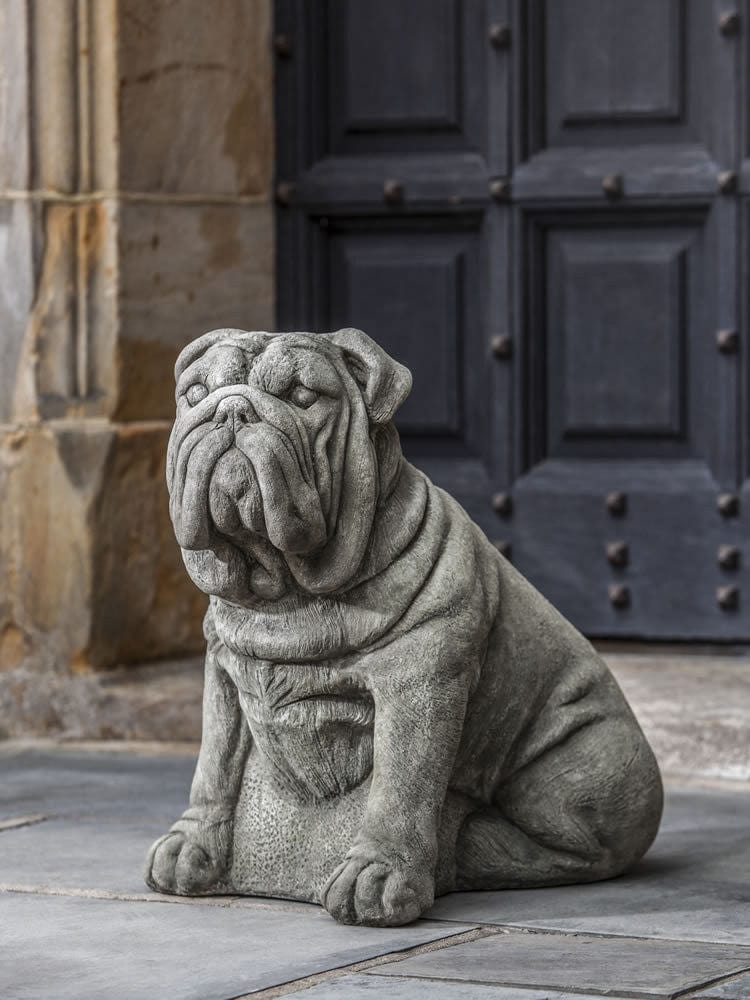The image is a vertically aligned rectangular photograph featuring a small stone bulldog statue with very droopy cheeks, ears, and rolls of fat on its body. The grayish-white statue is seated on dark gray stone tiles, facing slightly to the left but looking forward. Behind the statue, there is a robust, navy blue wooden door with multiple metal notches for decoration, hinting at a heavy and possibly steel-reinforced structure. To the left of the door is a weathered and chipped tan stone column. The entire setting is outdoor, with a concrete ground extending into the background, providing a sense of the statue's placement within a sturdy, aged architectural environment. There is no border or text around the image.